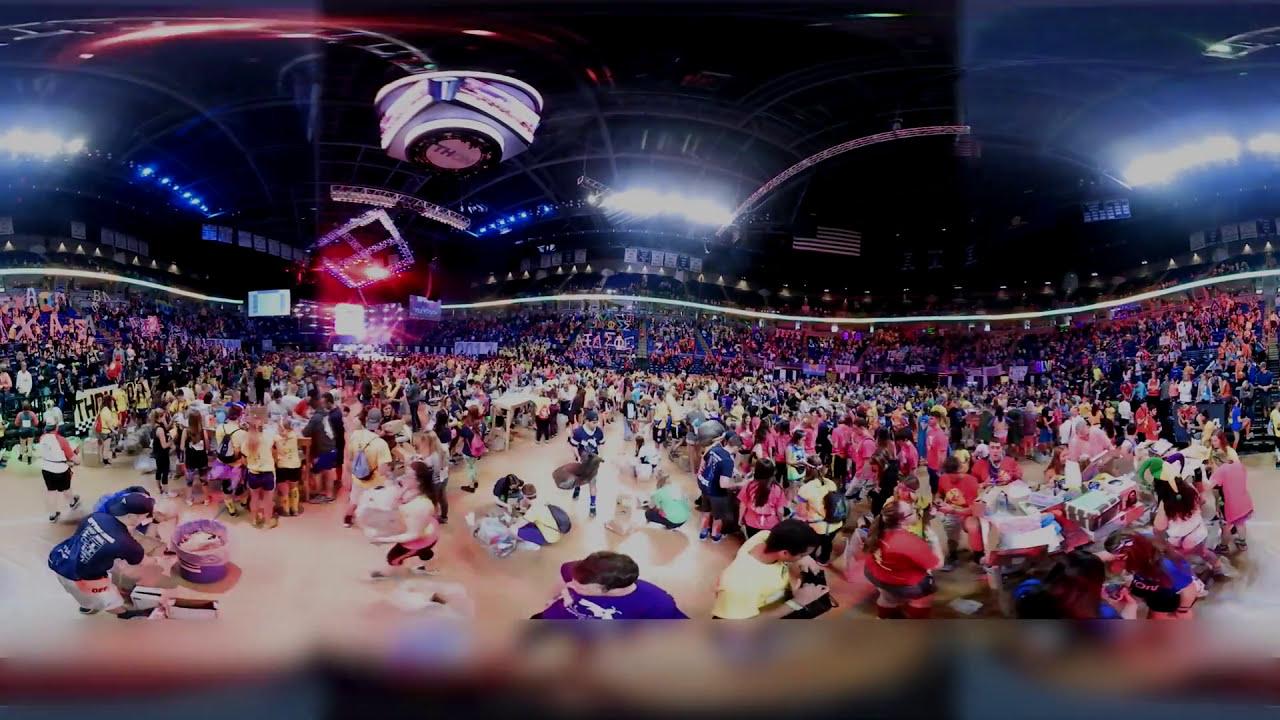The image depicts a bustling scene inside a large indoor Coliseum or convention center, characterized by its beige tile floor and massive arched ceiling. A prominent American flag and a scoreboard are visible, indicating the grand scale of the arena. Hundreds, possibly thousands, of people are spread throughout the venue, with many congregating around tables displaying various trinkets and exhibits. In the foreground, numerous attendees wear pink or red shirts, and one individual sports a distinctive Joker hat. The crowd, which includes both adults and children, some of whom are in costume and holding stuffed animals, has a lively and vibrant atmosphere. Among the swarming masses, people are seen carrying packages and engaging with different stalls. In the background, spectators fill the bleachers, and some individuals hold up large pink letters and Greek symbols, adding to the festive ambiance. Despite the absence of a specific event or sports game, the diverse throng of people and the myriad of activities convey the sense of a large-scale gathering, possibly an anime convention or a similar event.